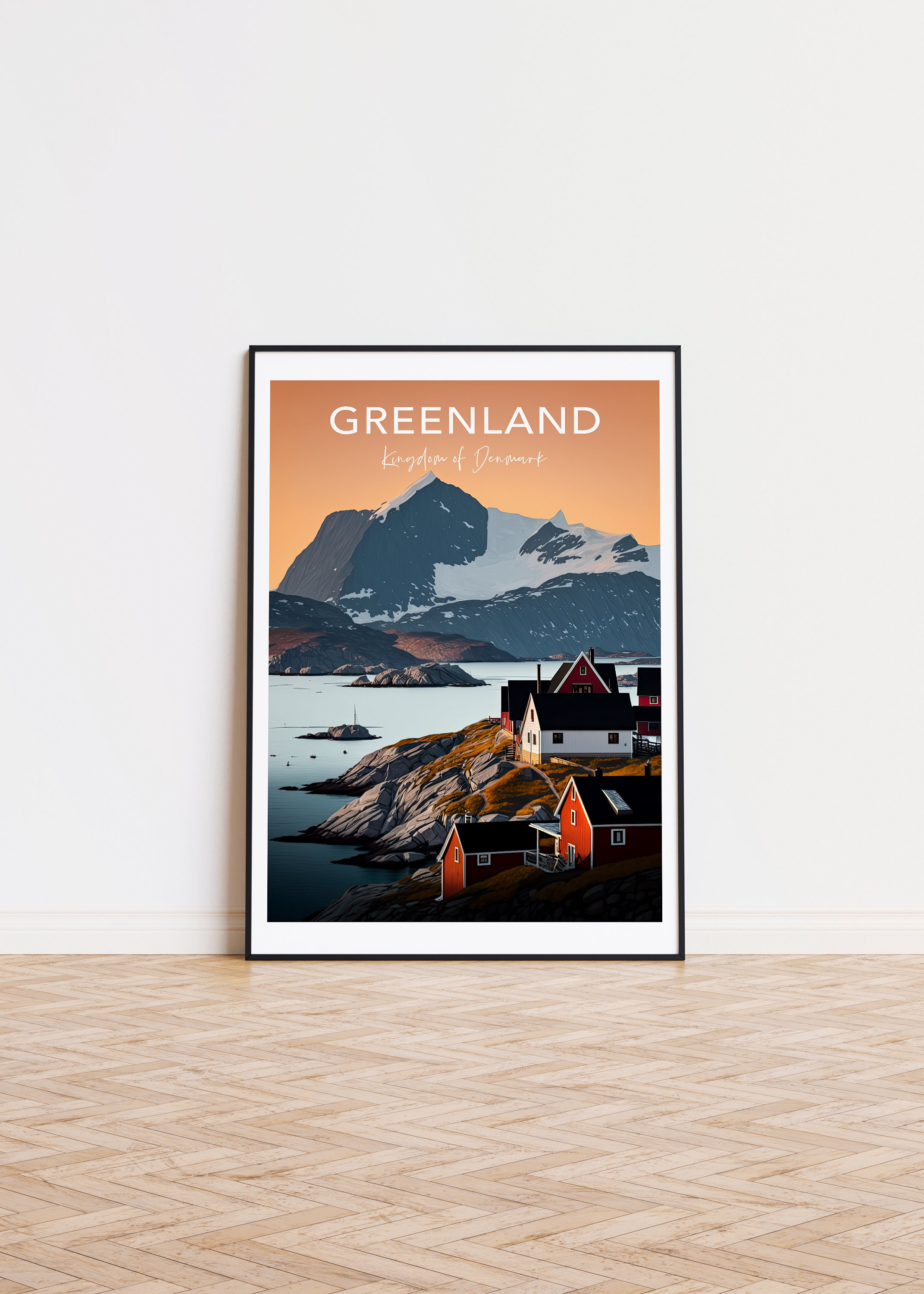This image features a large framed poster propped against a light gray or off-white wall. The floor is characterized by a complex pattern of light and dark tan bricks. The poster itself is encased in a very narrow black frame with a white border and depicts a picturesque coastal scene.

Centered in the poster is a charming cluster of white and red framed buildings, each one or two stories tall, with black roofs. These structures are perched on a rocky seashore, and in the background, across the water, lie majestic snow-capped mountains. The serene lagoon of the Arctic Ocean completes the idyllic landscape. At the top of the image, bold uppercase text reads "Greenland," with a smaller, cursive line below that likely says "Kingdom of Greenland" though the latter is difficult to distinctly read.